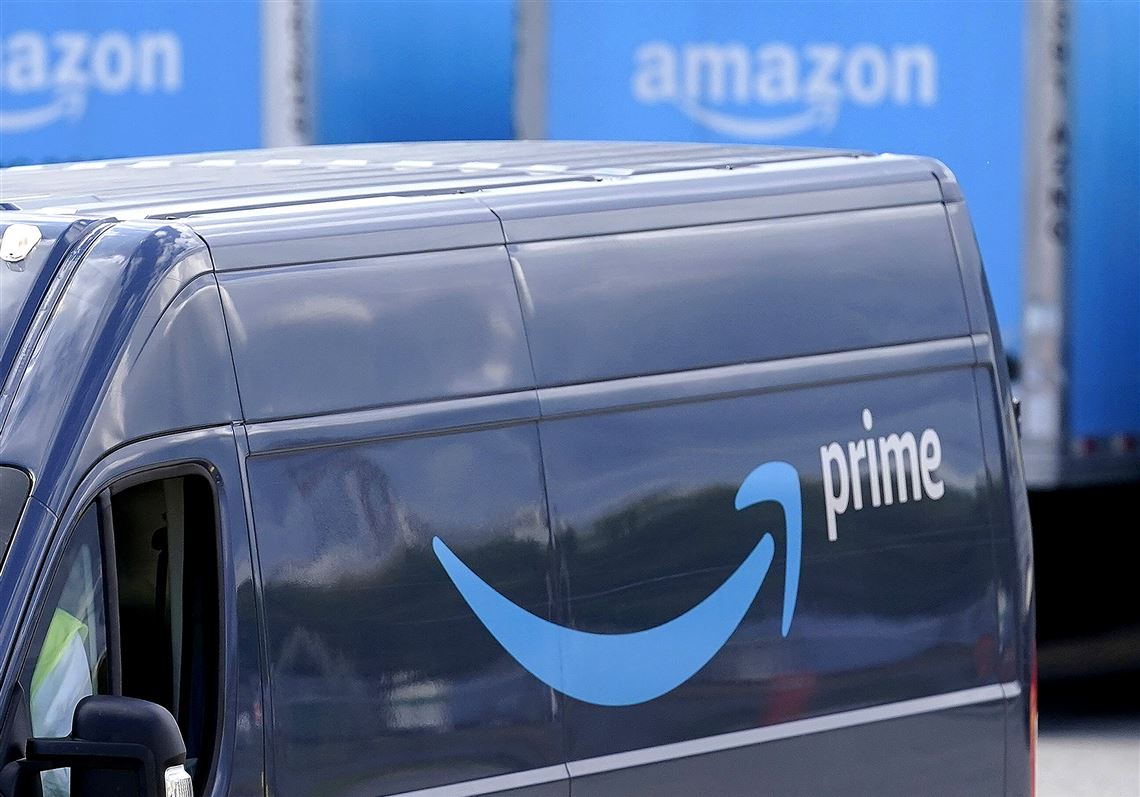We are looking at a remarkably sharp and clear photograph, likely taken from a screenshot, featuring an Amazon Prime delivery van. The van is painted in the familiar dark grayish blue color, adorned with a light blue swipe and the distinctive white Prime logo in lowercase lettering. The van is parked at an interesting angle, prominently positioned in the foreground. 

In the background, we see a row of tractor trailers meticulously backed into loading and unloading docks at an Amazon hub facility. The trailers, artfully out of focus, provide a contrasting backdrop that enhances the clarity and detail of the delivery van in the foreground. This composition beautifully illustrates the Amazon Prime delivery process, from large transport trucks to the final delivery vehicles. The photograph masterfully captures the essence of Amazon's logistics, merging the industrial scale of the hub with the more personal scale of the delivery service.